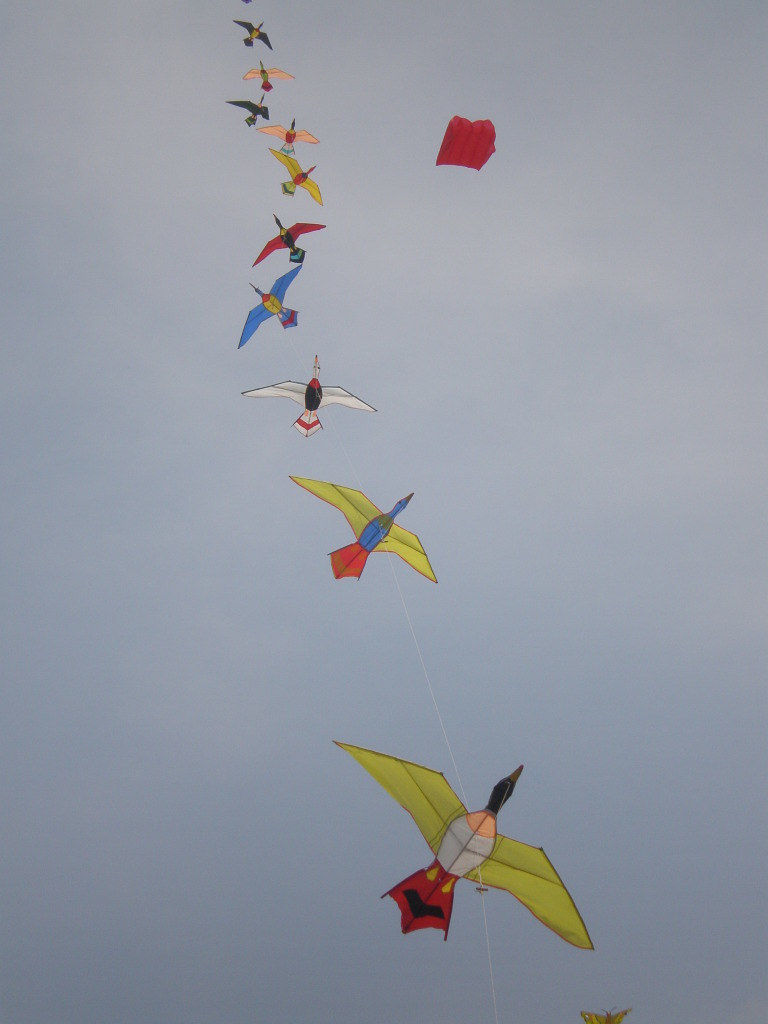This photo, taken from a perspective beneath the kites, captures a striking scene of 10 to 11 bird-shaped kites soaring into a mostly cloudy sky. The kites, strung along a single line of twine, give the illusion of colorful birds floating in the air with their wings beautifully spread out. The birds feature various colors, including yellow wings with blue bodies, white wings with black bodies, and other multicolored combinations. Despite a backdrop of fine mist-like clouds with hints of blue sky, the vibrant colors of the kites stand out vividly. Alongside these bird kites, a solitary red square kite can be seen in the distance, adding a unique element to the composition.